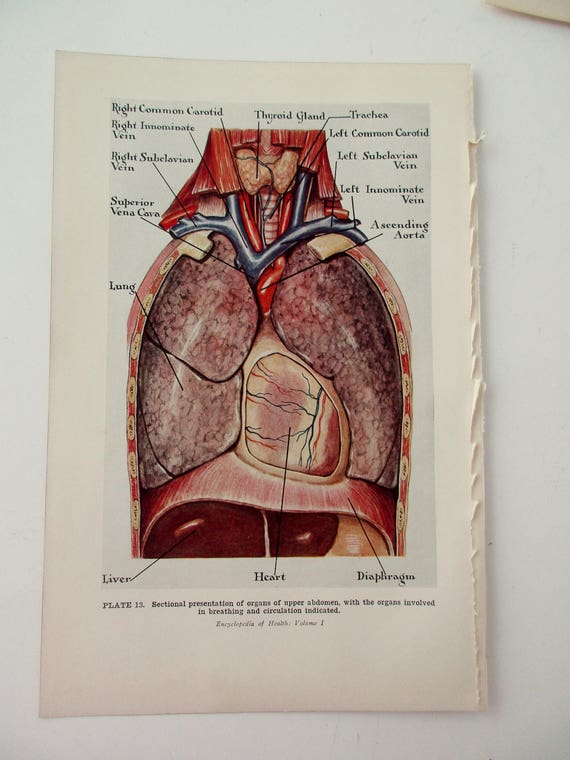This image depicts a highly detailed, colored anatomical illustration torn from a book, presumably an old anatomy atlas or medical magazine. The illustration showcases the esophagus, heart, lungs, thyroid gland, trachea, diaphragm, and liver. Notably, it focuses on muscles, veins, and organs rather than skeletal structures, providing a vivid, almost red meaty texture to the painted parts. Each anatomical component is meticulously labeled, including the right and left carotid arteries, right and left subclavian veins, and the ascending aorta, among others. The background of the page has a slightly yellowed, off-white appearance, indicating its age. The page bottom text reads, "Plate 13: Sectional presentation of organs of upper abdomen with the organs involved in breathing and circulation indicated." The right-hand side of the page shows clear rippling from where it was torn, adding to the historic and tactile quality of the image.